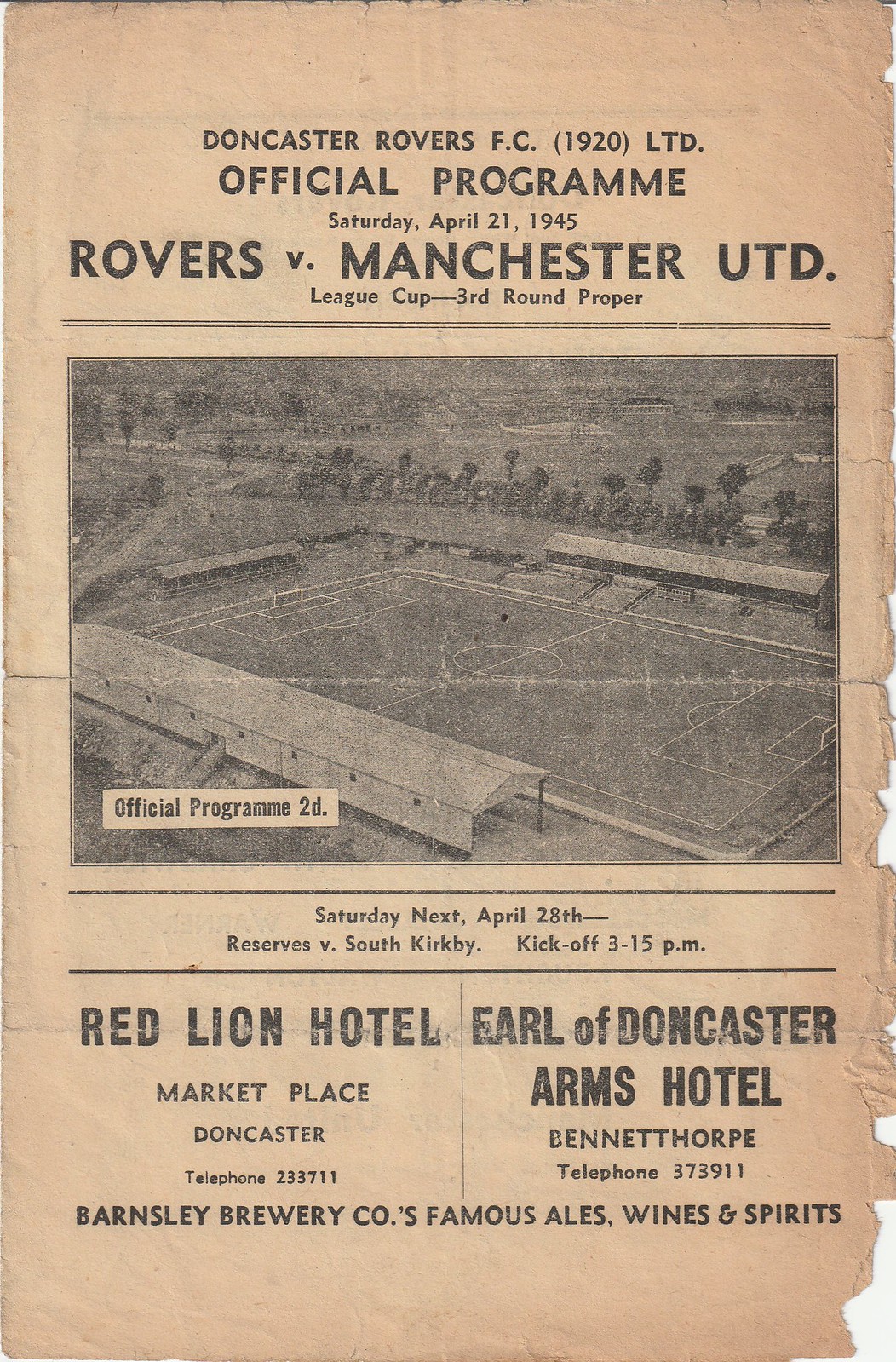The image depicts an aged, yellowed, and somewhat frayed official program for a Doncaster Rovers FC match against Manchester United in the League Cup third round proper, held on Saturday, April 21, 1945. At the top, the title reads “Doncaster Rovers FC Limited Official Program.” A black and white photograph of a soccer field with stadium bleachers and a backdrop of trees occupies the middle of the page. Below this, announcements indicate a reserves match against South Kirkby on Saturday, April 28, at 3:15 p.m. The bottom of the page features advertisements for the Red Lion Hotel in the Marketplace, Doncaster, with the telephone number 233711, and the Earl of Doncaster Arms Hotel in Bennet Thorpe. Additionally, there is a mention of Barnsley Brewery Co's famous ales, wines, and spirits.